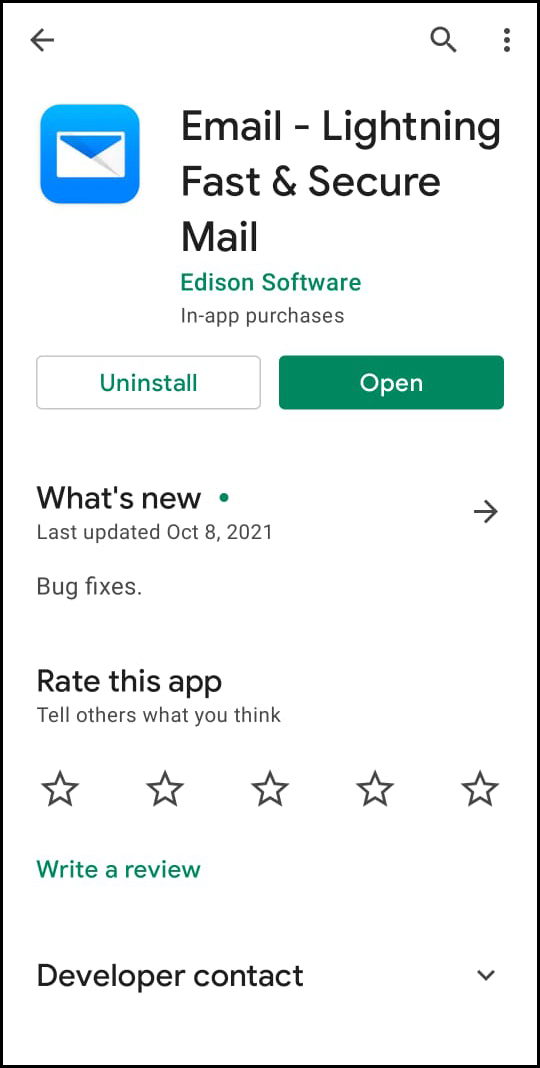This image depicts a detailed user interface of an app page. It features a rectangular-shaped box with a black border, oriented vertically. In the top-left corner, there is a black arrow pointing to the left. On the top-right corner are three icons: a magnifying glass, three vertical dots, and an envelope icon enclosed in a blue box. To the right of the envelope icon, black text reads "Email – Lightning Fast and Secure Mail," with green text below that stating "Edison Software". Below this, black text says "In-app purchases".

Further down, there is a white button labeled "Uninstall" written in green, beside a green button labeled "Open" in white. 

Following this section, the text "What's New" is displayed, under which the last update date is given as "Last updated October 8, 2021". Beside this information is a right-pointing arrow and the words "Bug fixes".

The next section invites users to rate the app with the prompt "Rate this app: Tell others what you think," accompanied by five stars. Below this, green text reads "Write a review". Finally, at the bottom, black text says "Developer contact".